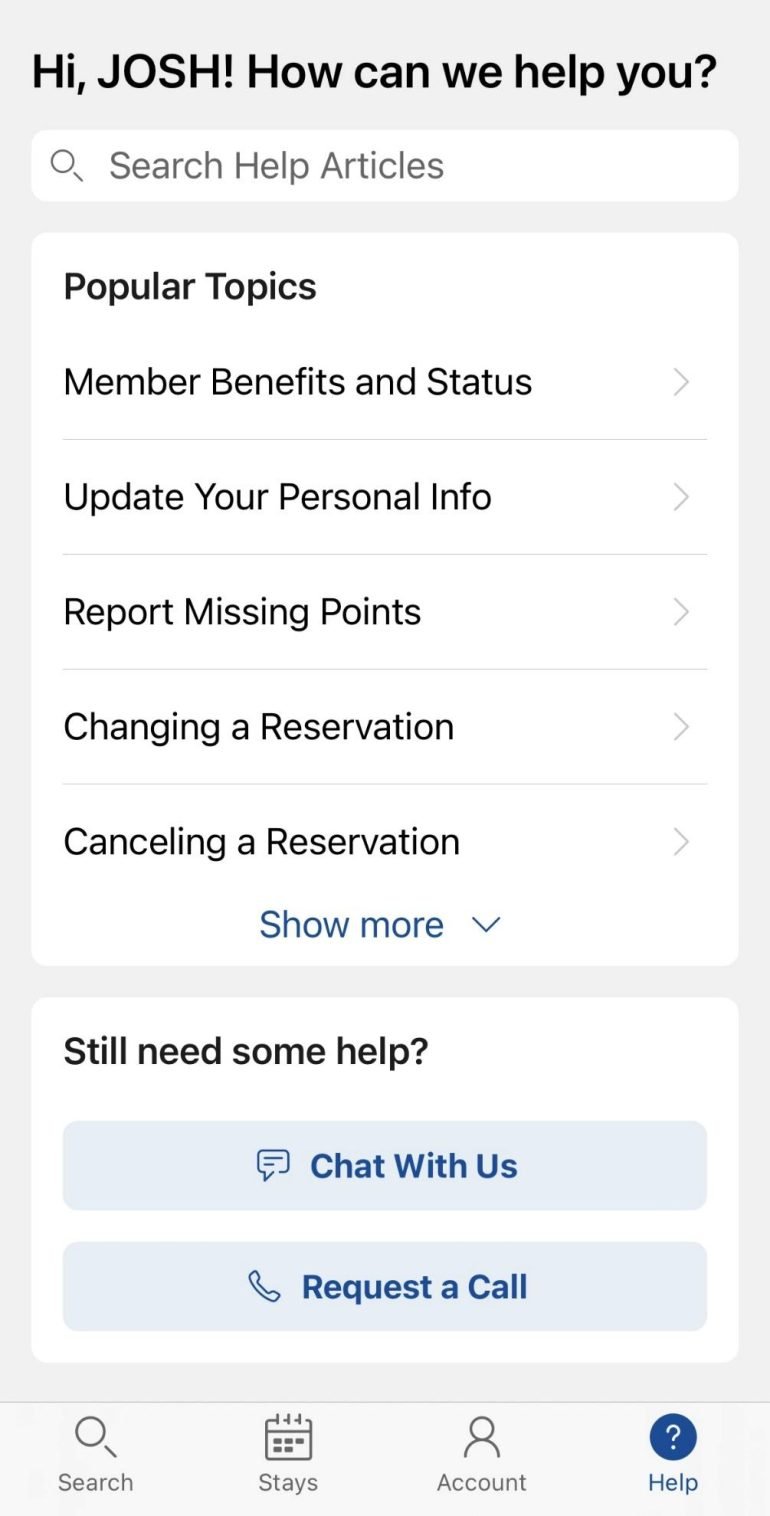A detailed and cleaned-up caption for the image could be:

"This portrait-format color screenshot captures a smartphone interface where a user named Josh is interacting with a help section on a website. The screen displays a friendly greeting, 'Hi Josh! How can we help you?' with a prompt to either type into the search bar at the top to search help articles or choose from popular topics listed below. The options available include 'Member benefits and status,' 'Update your personal info,' 'Report missing points,' 'Change a reservation,' 'Cancel a reservation,' with a 'Show more' arrow indicating additional topics that are not currently visible. For further assistance, two buttons at the bottom offer the choices to 'Chat with us' or 'Request a call.' The bottom navigation bar of the phone displays icons for 'Search,' 'Stays,' 'Account,' and 'Help,' although it is not clear which option Josh has selected."